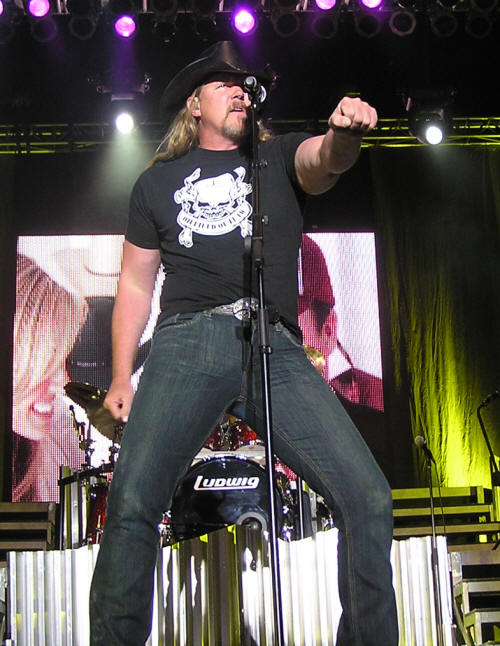The color photograph, captured in a portrait orientation, showcases a dynamic country performance on stage. The focal point is a male singer, who exudes energy with his left fist extended toward the viewer and his right hand also clenched by his side. He is adorned in classic country attire: a black cowboy hat, a black short-sleeve t-shirt featuring a white skull graphic surrounded by a ribbon, blue denim jeans, a brown leather belt, and an oversized, silver oval-shaped belt buckle. His long blonde hair and neatly trimmed beard and mustache complement his rugged look. 

Positioned at the center stage, he sings into a black microphone, held by a black stand, pointed towards his face. His eyes glance slightly upward and to the top right corner of the image, engaging with the performance. Behind him, a drum set rests on an elevated platform, framed by purple and white stage lighting. Adding a narrative element, a projection on the backdrop displays an image of a woman with blonde hair, smiling at an unseen man beside her, partially obscured by the singer. The overall style of the photograph is representational realism, vividly capturing the scene's authenticity.